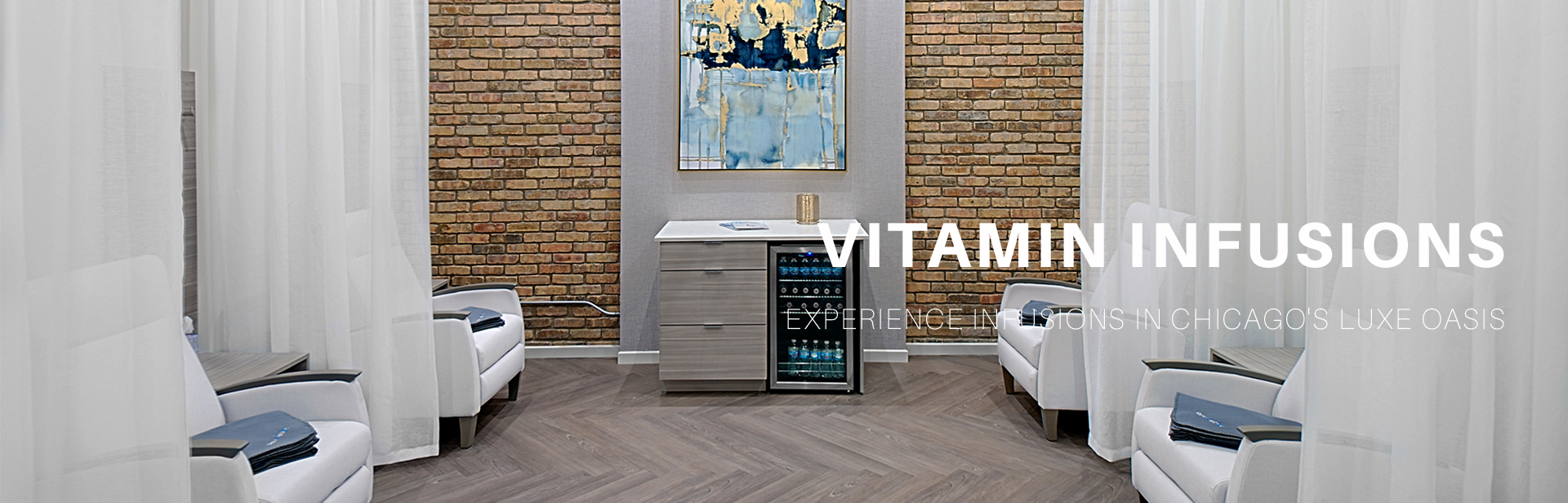This is a detailed color photograph of a spa treatment facility advertising vitamin infusions at Chicago's Lux Oasis. The image features large, bold, all-capital letters in white that read "VITAMIN INFUSIONS." Directly beneath it, in smaller, faint white letters, it says, "Experience Infusions in Chicago's Lux Oasis." The setting is visually striking, divided into sections by tall, sheer white curtains, which offer optional privacy for guests receiving treatments. 

Central to the image is a gray wall adorned with a vibrant artwork in hues of teal, gold, and dark blue. Directly in front of this wall is a glass-windowed cabinet or case, presumably storing various vitamins and infusion products. Flanking the gray wall are symmetrical brown brick walls that add a rustic contrast to the modern interior. 

On each side of the central display, there are two white leather recliner chairs, making a total of four, arranged in pairs. Each chair is prepared for comfort, with gray blankets folded neatly on the seats and an additional cushion possibly intended for lower back support. Placed on the chairs are blue folders, suggesting informational packets or menus for the treatments offered. The clean, organized arrangement, along with the soothing color palette and comfortable seating, underscores the serene and luxurious experience promised by this spa.